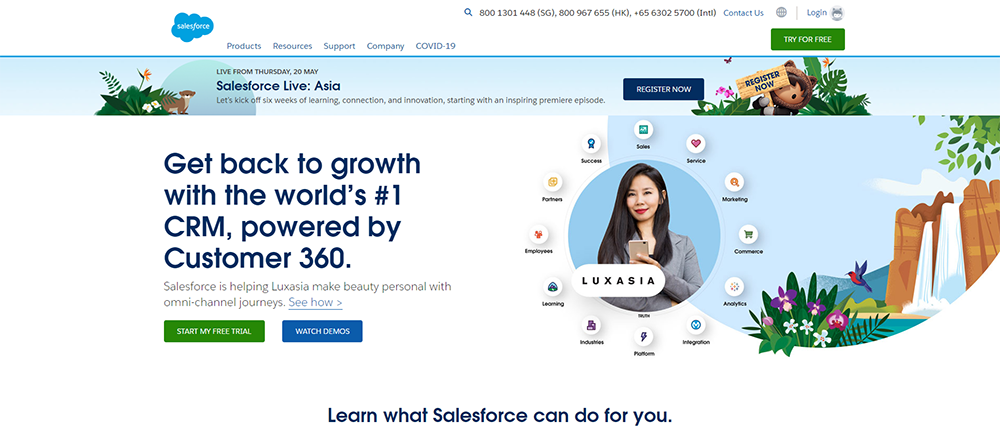The screenshot depicts the homepage of a website designed with a rectangular layout, where the width is significantly greater than the height. At the very top, there is a white banner stretching horizontally across the entire width of the page. On the left side of this banner, a blue cloud icon with white text that reads "Salesforce" is prominently displayed. To the right of the cloud icon, a series of clickable options are listed in blue text: "Products", "Resources", "Support", "Company", and "COVID-19".

Towards the center-right of the banner, a series of contact numbers are presented in black text: "800-1301-448-SG, 800-967-655-HK, +65-6302-5700, International". Adjacent to these numbers, blue text reading "Contact Us" provides a direct interaction point for user inquiries. Following this, a small gray globe icon is displayed, next to which "Login" is written in blue text. Beneath the "Login" text, a green rectangular button with white text offers a "Try for Free" option.

Immediately below this white banner, a thin blue line runs horizontally across the page, creating a visual separation from the light blue banner below it. On the right side of this secondary banner, a cartoon illustration features a brown otter with a tan stomach emerging from a green bush, which has an orange flower blooming atop it.

This detailed structure of the homepage is designed to provide clear navigation and quick access to various features and support options, while the friendly otter illustration adds a touch of whimsy to the user experience.